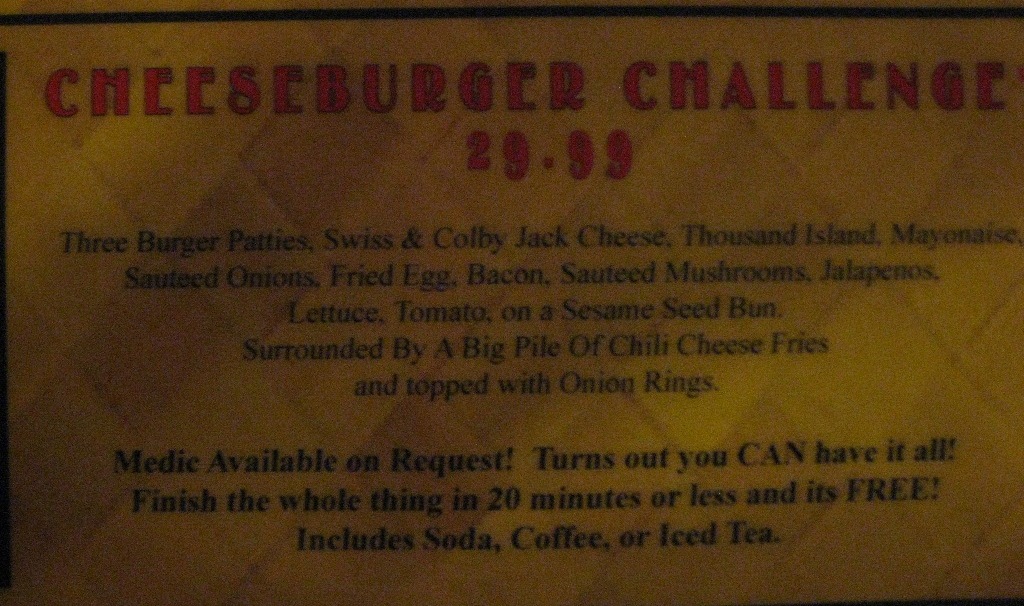The image depicts a vintage-style menu item on the back page of a menu. The background is a darker yellow with triangular patterns framing the edges. At the top, "Cheeseburger Challenge - $29.99" is prominently displayed in large red letters. Below it, the detailed description is written in small black text. The challenge consists of three burger patties topped with Swiss and Colby Jack cheese, Thousand Island dressing, mayonnaise, sautéed onions, a fried egg, bacon, sautéed mushrooms, jalapeños, lettuce, and tomato, all assembled within a sesame seed bun. Accompanying this colossal burger is a generous serving of chili cheese fries, crowned with onion rings. 

In slightly larger black letters, it humorously states, "Medic available on request!" The text explains that if one manages to consume everything within 20 minutes or less, the meal is free and includes a beverage choice of soda, coffee, or iced tea. This single-page menu item stands out due to its detailed and tempting description, accompanied by a humorous and challenging appeal.